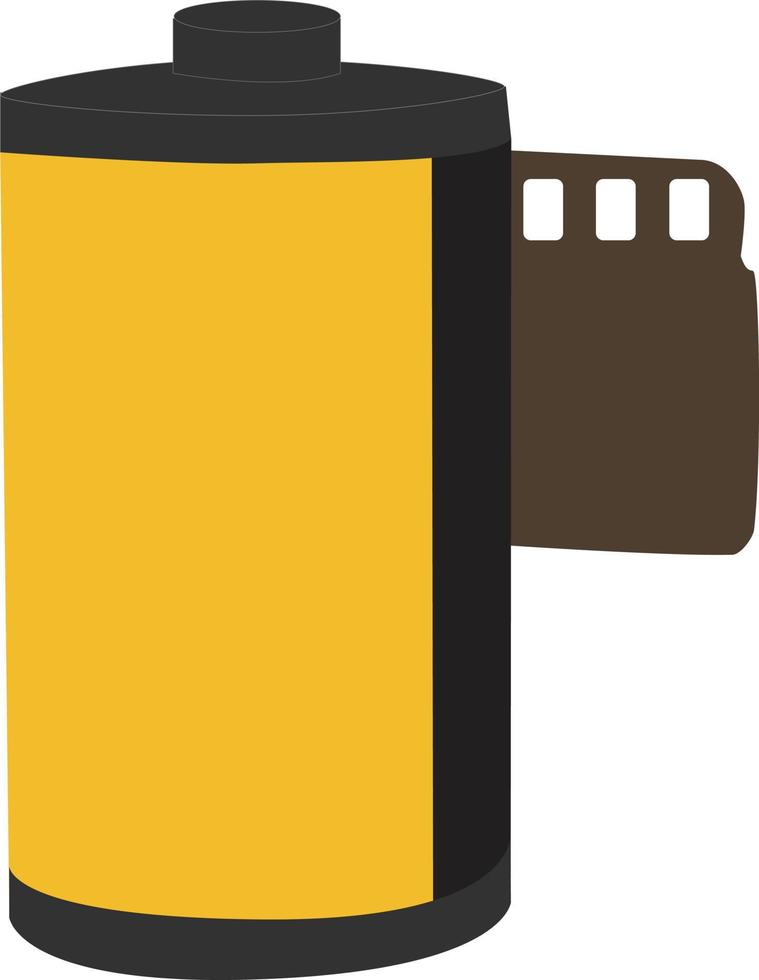The image depicts a highly enlarged, computer-generated 35mm film canister against a white background. The canister itself is predominantly black with a plain yellow label on the front, devoid of any branding or text. A round, black lid is situated at the top of the cylinder. Emerging from the right side of the canister is a strip of brown film, featuring three perforated holes along the top edge and a side notch, details typical of 35mm film ready to be fed into a camera. The film strip protrudes in such a way that it reveals the white background through its cutouts. The overall depiction emphasizes the oversized nature of the canister and its components, highlighting the black and yellow color scheme and the detailed features of the film strip.